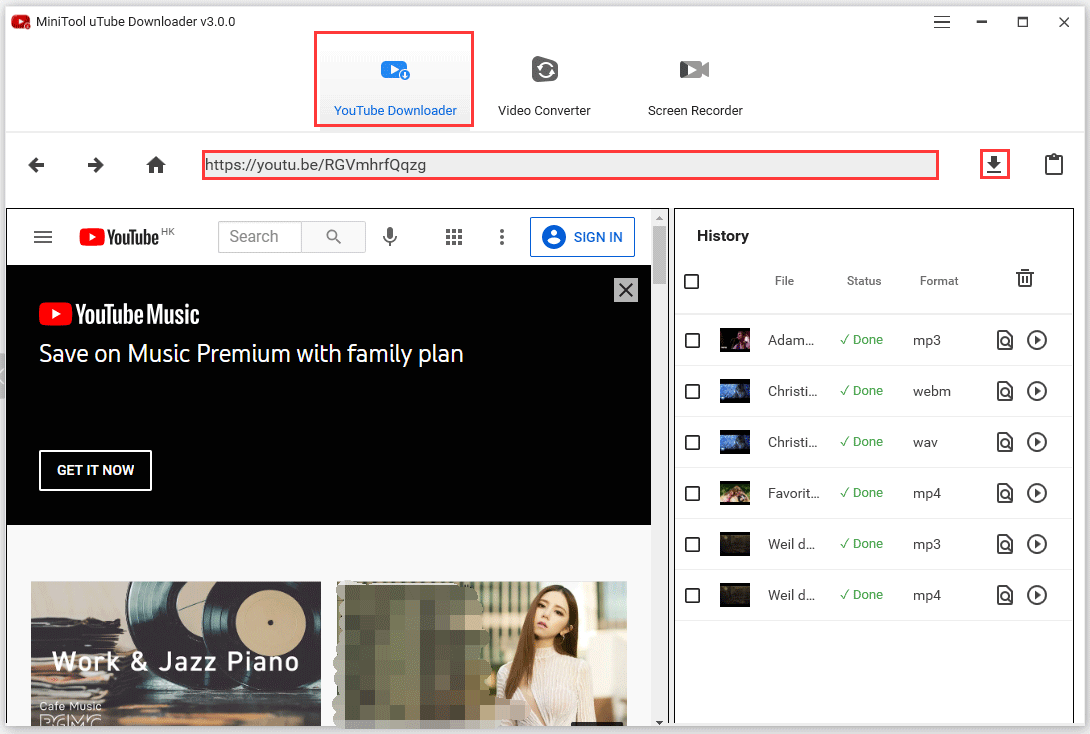Screenshot of the YouTube Downloader Web Page

The image is a screenshot of the MiniTool YouTube Downloader Version 2.0.0 web page, hosted on what appears to be YouTube’s platform or a related site. The page predominantly features a white background. In the top left corner, the recognizable YouTube logo is displayed alongside the text "MiniTool YouTube Downloader Version 2.0.0". 

On the top right of the page, there are four distinct icons arranged horizontally: the first icon shows three horizontal lines, the second represents the minimize action, the third is the maximize page icon, and the fourth is an 'X' indicating the exit functionality.

Beneath this header, three horizontal boxes are aligned. The first box, outlined with a red border, features a blue YouTube logo and the text "YouTube Downloader" in blue. The second box has no border and contains black text that reads "Video Converter" along with an icon depicting a file with circular arrows. The third box also lacks a border and bears the text "Screen Recorder" beside an icon of a video camera with a play button.

Another address bar, surrounded by a red border, sits directly below these boxes, flanked on the left by left and right navigation arrows and a home icon. Further down is another YouTube logo, a search bar, and an option to sign in.

A prominent black box further down features white text that reads "YouTube Music." Below this, the text "Save on Music Premium with Family Plan" is shown. Adjacent to this section, a white-bordered box displays the call to action "Get It Now."

To the right is a vertical series of elements under the header "History," featuring approximately seven checkboxes, each representing a different video download. Small thumbnails accompany each entry, with partial text descriptions and a green text status "Done" beside each.

Finally, just below the black YouTube Music box, two additional boxes are displayed: one labeled "Work in Jazz Piano" with a background image of records, and the other featuring a picture of a woman.